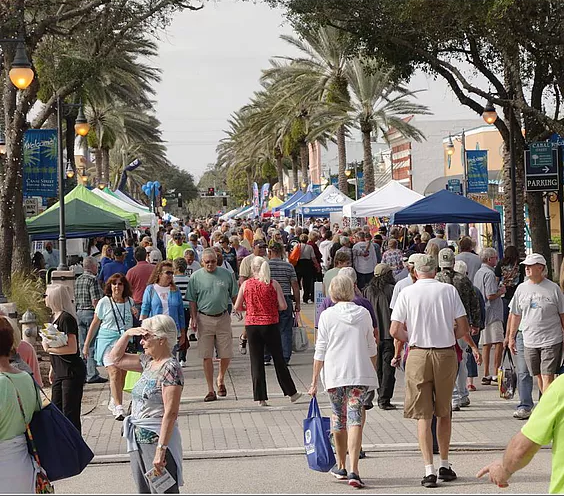The image depicts a bustling outdoor street fair in an area with a tropical climate. The street is densely packed with people of all ages, many dressed in shorts and short sleeves, carrying bags, and shading their eyes from the daylight sun. Numerous booths with blue, white, and green canopy tents line both sides of the street, with blue and white tents on the right and green and white canopy tents on the left. Behind the rows of booths are storefronts and buildings, with light posts adorned with banners. Tall palm trees stretch along both sides of the street, from the foreground to the horizon. The sky appears overcast, and power lines are visible in the distance. The street, likely blocked off for the event, is filled with people walking and shopping, creating a vibrant market atmosphere.